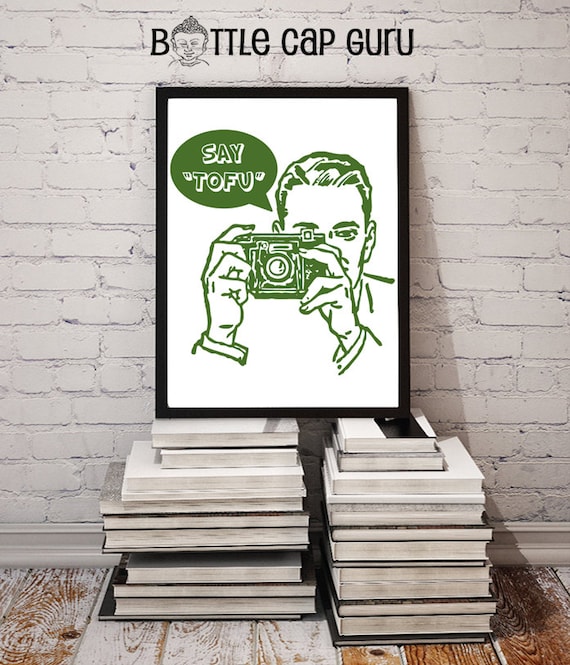The image features a large framed poster perched atop two stacks of white books, leaning against a whitewashed brick wall. The stacks of books, positioned on a whitewashed wooden floor, face different directions—one with its spines against the wall, the other with its spines facing towards the first stack. The black-framed poster has a vibrant yellow background with black graphics. It showcases a caricature of a man using an old-fashioned camera, accompanied by the text "Say Tofu." Additionally, the words "Bottle Cap Guru" appear above the man's illustration, with the "O" in "Bottle" stylized to resemble a child’s face. One of the white books includes a noticeable black accent.